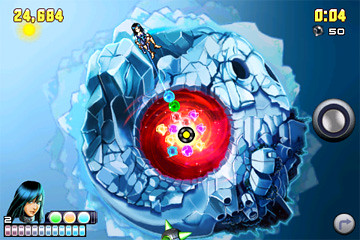A screenshot from a video game, possibly an anime-inspired artistic work, showcases an intense scene. In the top-right corner, a countdown timer displays the number '4'. The centerpiece of the image is a looming gray asteroid-like structure against a blue background. The interior of this structure glows bright red and is filled with an array of multicolored jewels. A character, whose precise actions are unclear, appears to be navigating towards the vibrant core. The overall aesthetic of the game includes blue-hued numbers and interface elements, contributing to the futuristic and high-energy atmosphere of the scene.